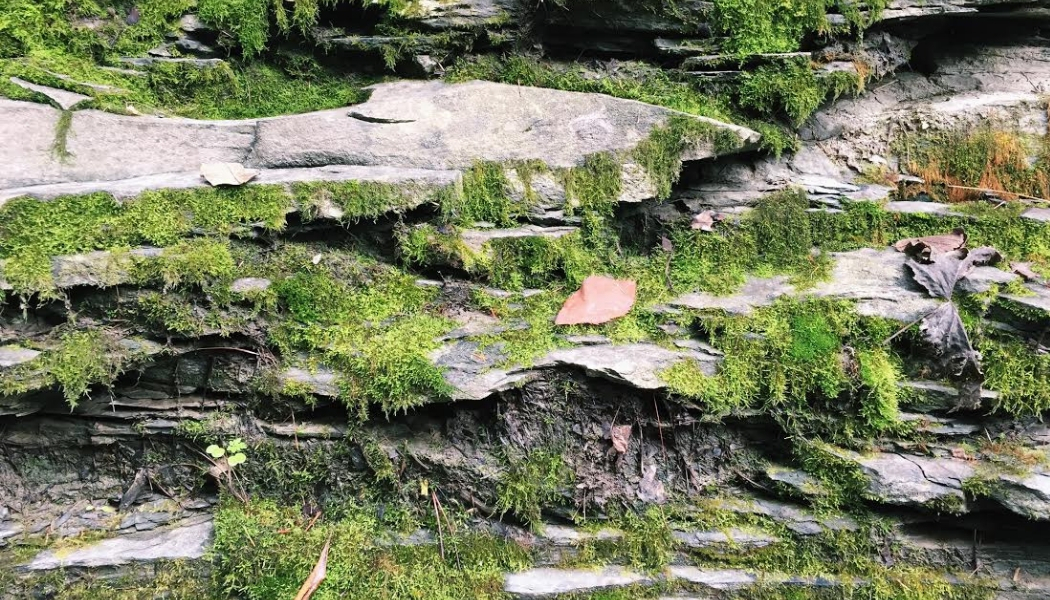The image captures a striking natural stone wall composed of an array of light-colored, shelf-like limestone strata interspersed with darker gray sections, giving it a uniquely rugged and etched appearance likely shaped by erosion. Verdant greenery, including hanging ferns, moss, and lichen-like plants, cascades down the cliffside, adding a vibrant contrast to the rock’s muted tones. Enveloped in this lush vertical landscape, the small signs of life and decay can be spotted—rust-colored flowers, dying leaves, and sticks—nestling within the crevices and the flat-lying rocks at the base. Amidst the greenery, a small, enigmatic cloth-like element garners curiosity, its nature indeterminate, blending seamlessly into this serene, untouched nature refuge.